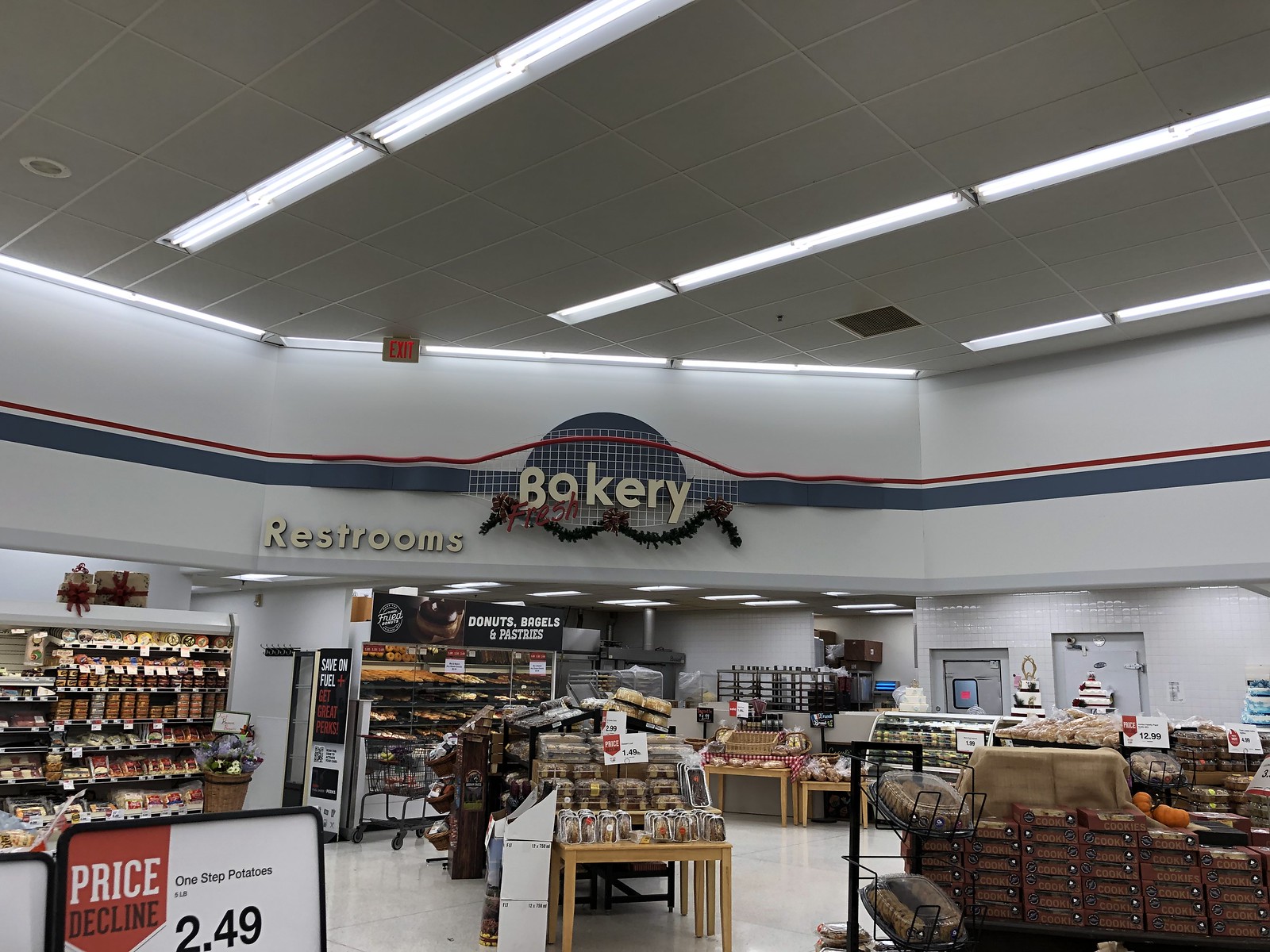The photograph captures the bustling interior of a grocery store, specifically focusing on the bakery and surrounding sections. Dominating the back wall, the word "Bakery" is prominently displayed in white lettering against a dark background. Above "Bakery," there is a noticeable red element, likely a light or decorative feature. Adjacent to the "Bakery," the word "Restrooms" is clearly marked in white letters on a white background.

The bakery section is adorned with festive foliage, possibly holiday decorations, enhancing its inviting atmosphere. Various breads and an assortment of cakes are meticulously arranged; the cakes, packaged in brown boxes, are stacked high to the right. Centrally located within the bakery area, an assortment of breads is displayed on tables alongside other baked goods, though the exact items are unclear.

To the right side of the image, a deli section is visible, displaying an array of luncheon meats in a refrigerated case—convenient for customers to peruse and select. In the foreground, a visible price tag of $2.49 draws attention, situated towards the left. Other signage includes "Donuts" and "Bagels," adding to the comprehensive overview of the bakery offerings. This photograph vividly encapsulates a snapshot of the grocery store's bakery area, brimming with diverse baked goods and deli items.